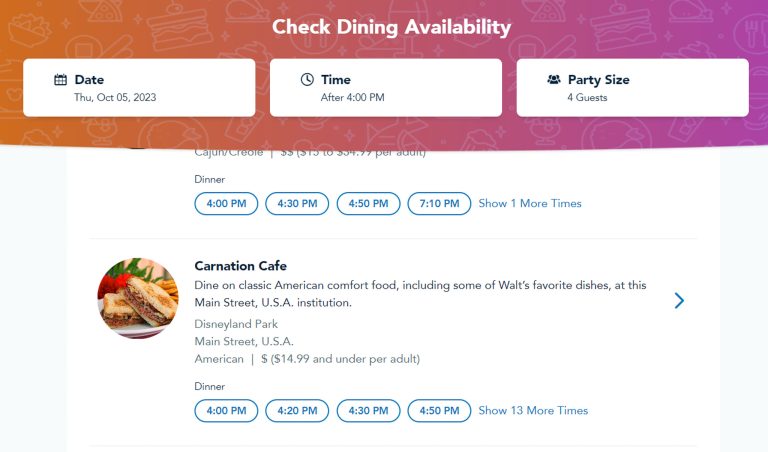The image is a screen capture from a desktop application page dedicated to dining reservations. At the top, there is a prominent banner featuring a gradient that transitions from orange on the left to pink on the right. The banner displays the text "Check Dining Availability" in crisp white letters. 

Directly below the banner, the interface presents three primary options for checking availability. The first is a white rectangle with smoothly curved corners, displaying the current date: "Thursday, October 5, 2023." The second white rectangle indicates the time, showing "after 4 p.m." The third rectangle outlines the party size, specifically "for 4 guests."

Further down the page, additional time options are shown in vivid blue text within a white background oval, inviting the user to select their preferred dining time. Below these options, an enticing image of sandwiches arranged on a white plate can be seen. To the right of this image, the name "Carnation Cafe" is written in elegant black text.

The layout is designed for ease of use, with clear visual cues and a harmonious color scheme guiding the user's attention through the process of checking dining availability.